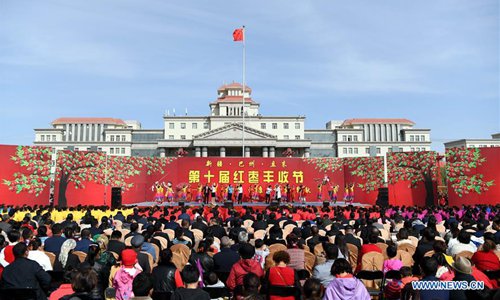The image is a detailed photograph of a public gathering in China, sourced from www.news.cn. Dominating the scene is a large, predominantly cream-colored and gray building with a symmetrical structure, featuring a central portion adorned with marble columns and flanked by flat, silver-gray extensions. The building's roofs are a striking red. Above the building, the sky is blue with thin, wispy white clouds.

Central to the image is a tall flagpole bearing the red Chinese flag, positioned towards the midpoint of the scene. In front of the building is a sizable stage with a vibrant red backdrop, showcasing yellow Chinese characters. The stage is adorned with painted green trees that have red fruits and pink flowers.

In the foreground, a large audience is gathered, densely packed and attentively facing the stage. Many individuals in the crowd are wearing red, and some appear to have their heads bowed. On the stage, performers in bright, multi-colored costumes, some adorned with flowers, are engaged in a performance. The overall scene captures a festive, cultural event with a significant emphasis on the crowd's engagement and the vivid cultural decor of the stage.